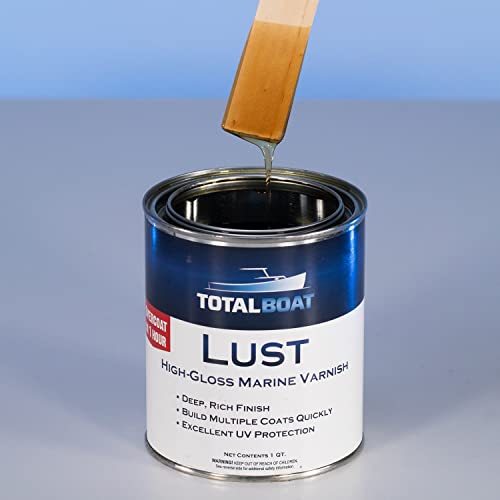In the image, a can of Lust High Gloss Marine Varnish from Total Boat sits prominently on a gray tabletop, against a blue wall background. The can is open, revealing a clear, glossy varnish inside from which a wooden paintbrush or stir stick drips the liquid back into the can. The can itself is primarily white with a distinctive blue band near the top, featuring an illustration of a boat and the brand name "Total Boat." The product name "Lust" is clearly labeled as a high gloss marine varnish. Descriptive text on the white portion of the can promises a deep, rich finish, the ability to build multiple coats quickly, and excellent UV protection. Additionally, a red banner is part of the can's design. The scene captures a moment of preparation, with the varnish ready to be applied, emphasizing both the quality and intended use of the marine product.